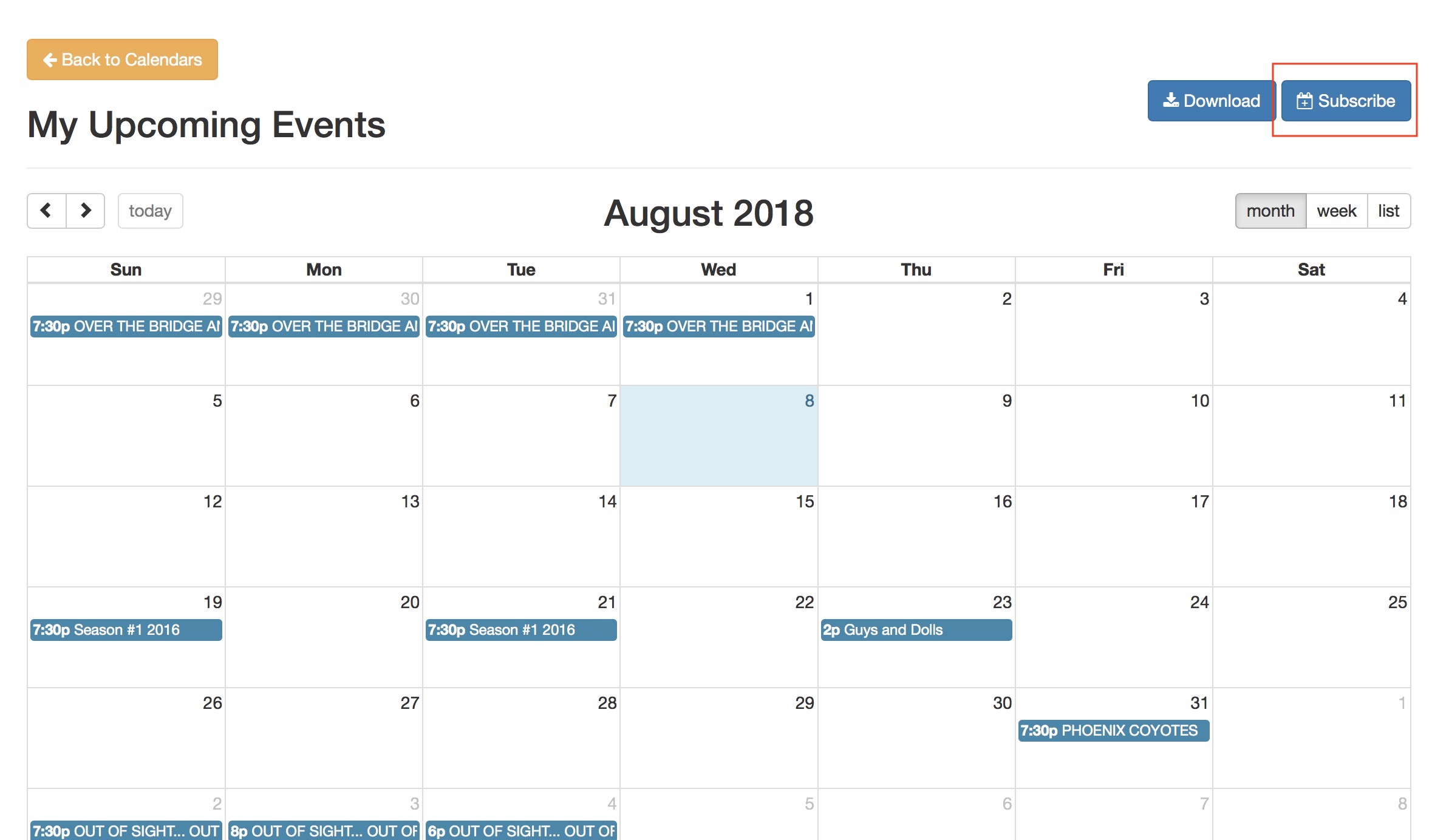This image is a detailed snapshot of an August 2018 calendar. The top left corner is titled "My Upcoming Events." Above this title, an orange button with white text and a left-pointing arrow reads "Back to Calendars." In the top right corner, there are two options: a download button and a subscribe button, which is outlined in red. The main calendar occupies most of the page and is oriented horizontally, spanning from Sunday to Saturday. It includes the dates for August and the final three days of July. Various events are listed across the calendar, including "Over the Bridge," "Guys and Dolls," "Out of Sight," "Season 1, 2016," and "Phoenix Coyotes," each accompanied by their respective times on the left.